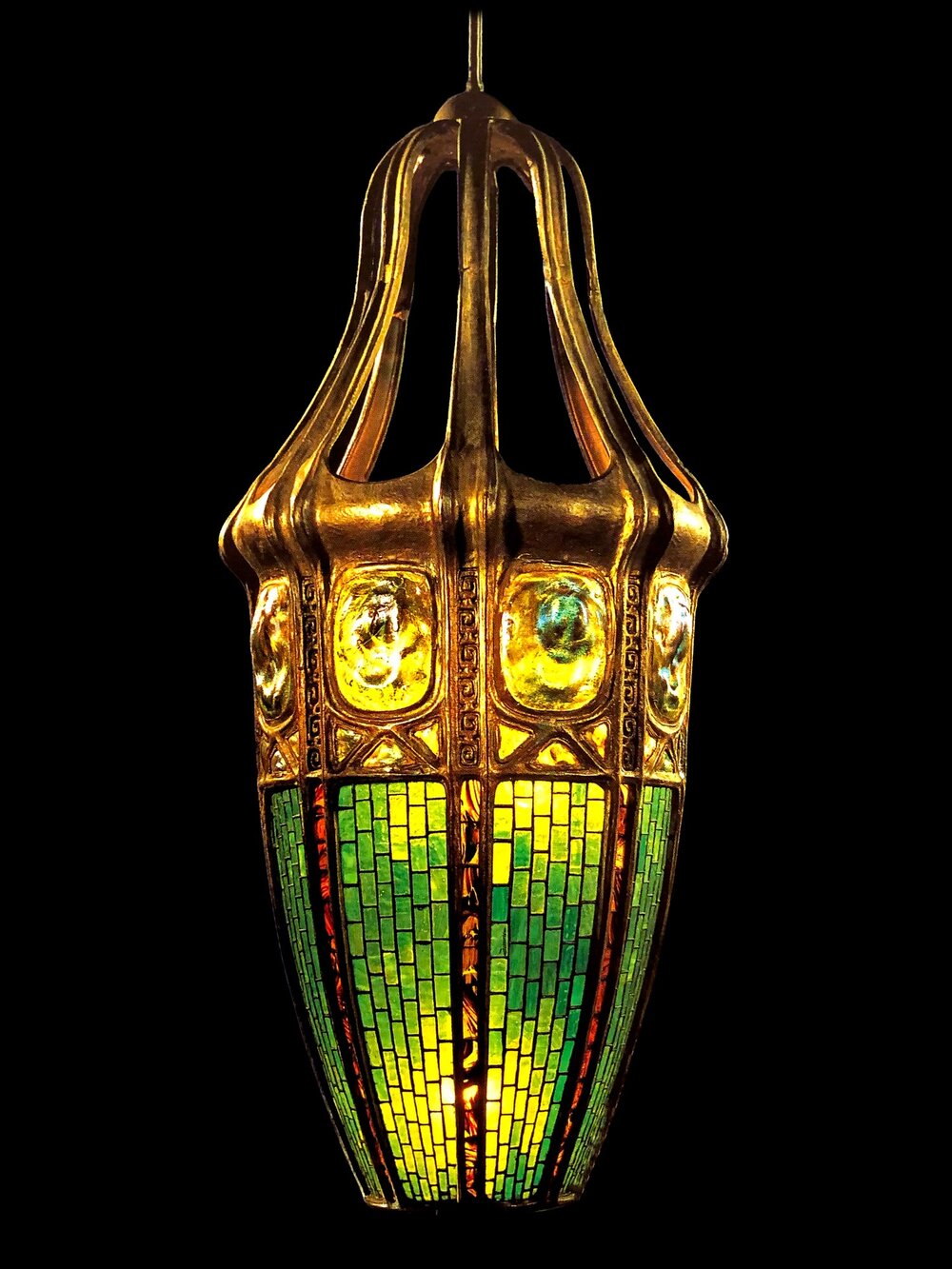The image features a close-up of an ornate lantern set against a completely black background. At the top of the lantern, there is an acorn-shaped or bell-like structure with intricate gold metalwork that exudes elegance. Moving downward, the sides of the lantern are adorned with a series of green, yellow, and amber-colored tiles that become smaller and more closely spaced as they approach the bottom. Between these tiles, there are striking red stripes with intricate red and yellow designs. The combination of gold at the top and the vibrant mosaic of colors running down the lantern makes it a visually captivating and classy object.